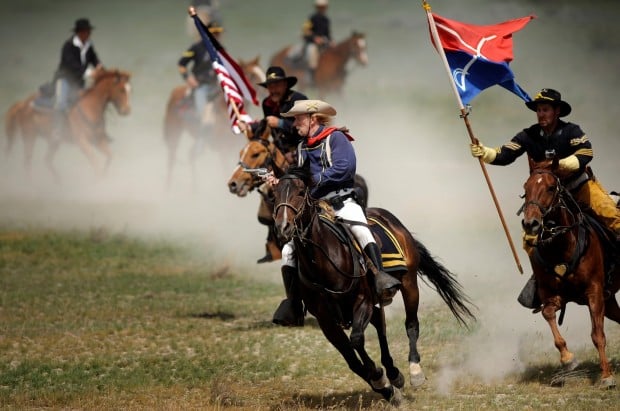Captured in this vibrant action shot is a thrilling rodeo scene featuring six men on horses galloping across an open field, their attire and demeanor reminiscent of colonial times. The foreground is dominated by three men racing towards the viewer, their dynamic movement kicking up a cloud of dust. The first rider, on a dark brown horse, proudly waves an American flag. He is distinguishable by his black brimmed hat, a mustache, and traditional rodeo attire consisting of a blue shirt, white pants, and black boots. To his right, another rider on a similarly dark brown horse holds a flag that is divided into a red upper section and a blue lower section, adorned with crossed scimitars. He complements his flag with a light brown, tri-cornered hat, a blue shirt, and a red bandana. The third rider in the foreground, mounted on a light brown horse, displays a similar sense of style with a white hat and denim clothing. The other three men in the background, though slightly out of focus, mirror the attire of their fellow riders and contribute to the overall spirit of the scene. The diversity in horse colors adds to the rich visual texture, ranging from dark brown to lighter shades. The collective imagery of men, horses, and flags set against the swirling dust captures the essence of a bygone era with a clear emphasis on tradition and action.